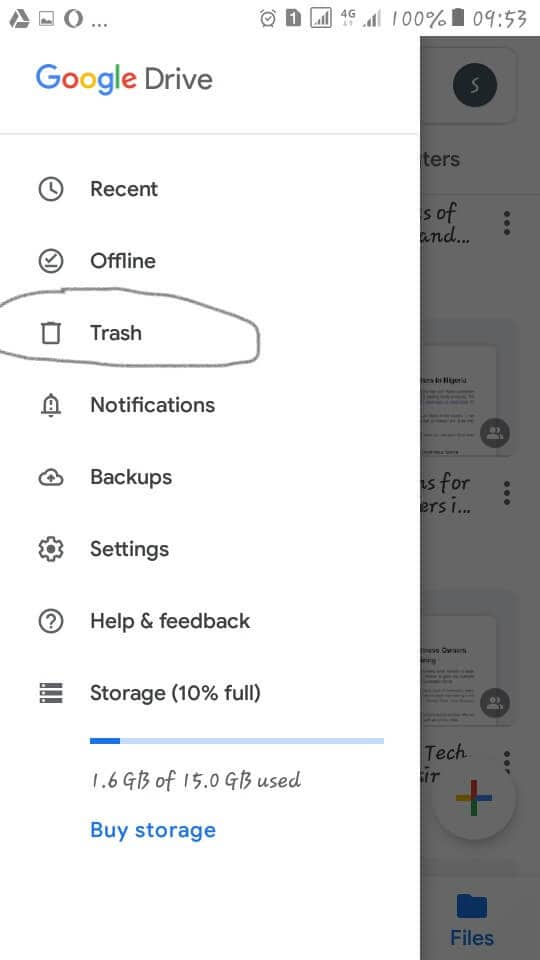Screenshot of a Google Drive App Menu

The screenshot displays the left-hand menu within the Google Drive app, showcasing a variety of features and options available to the user. 

At the top, the iconic Google logo is prominently displayed, with the letters colored as follows: a capital 'G' in blue, a lowercase 'o' in red, another lowercase 'o' in yellow, a lowercase 'g' in blue, a lowercase 'l' in green, and a lowercase 'e' in red. 

Following the logo, there is a capital 'D' in black for the word "Drive," with the remainder of the word also in black. 

A light gray horizontal divider separates the logo from the menu options below.

The menu options are listed sequentially as follows:

1. **Recent**: Accompanied by a clock icon.
2. **Offline**: Indicated by a circle with a checkmark inside and a horizontal line beneath. Notably, a hand-drawn circle highlights this option, which includes an image of a small black can.
3. **Trash**: Represented by a black trash can icon.
4. **Notifications**: Shown alongside a bell icon with a string attached.
5. **Backups**: Indicated by a cloud icon with an upward-pointing arrow.
6. **Settings**: Displayed with a gear icon featuring a dot in the center.
7. **Help & Feedback**: Associated with a circle icon containing a question mark.

At the bottom of the menu, the storage usage is detailed. There are three horizontal lines with a dot on the left of each, and the text reads "Storage 10% full." A progress bar extends across the menu, primarily light blue with a small darker blue section at the start. 

Below this, in an elegant font, it says "1.6 GB of 15.0 GB used." Underneath, the option to "Buy Storage" is highlighted in blue.